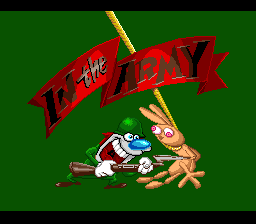This image, which appears to be a computer-generated screenshot resembling a title screen of a video game, features a scene with a strong "Ren and Stimpy" vibe. At the top, a red cartoon banner reads "In the Army" in a gray font. The art style is pixelated, framed by thin black strips at both the top and bottom edges, and set against a uniform green background.

Central to the image is a cartoonish figure with a big blue nose and a wide, toothy grin. This character closely resembles a dog dressed in a green army uniform, complete with a helmet, shirt, pants, and brown boots. It wields a rifle with a bayonet at the end, which is pointed at a hanged bunny rabbit. The bunny, suspended by a large yellow rope, has a peachy-brown color and exaggerated pink eyes, giving it an odd, crazy appearance.

The character's eyes are close together, and it has a manic expression, further enhancing the whimsical and slightly dark humor of the scene. The bunny is clearly lifeless, adding a stark, surreal touch to this cartoonish yet unsettling tableau.